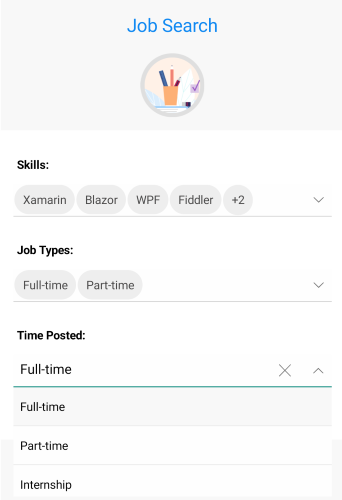The image features a light gray rectangular box at the top containing the text "Job Search" in blue. Below this, there is a circular icon displaying an illustration resembling a cup filled with markers and a pencil. Underneath the icon is a white area labeled "Skills," which includes several boxes listing skills such as Xamarin, Blazor, WPF, and Fiddler, with an additional note of "plus two" skills.

Beneath the skills section, there is a horizontal arrow pointing downward, followed by a line extending left to right. Below this line, the section is labeled "Job Types," featuring buttons for "Full-Time" and "Part-Time" options. Another arrow pointing downward appears, directing the viewer to a section labeled "Time Posting." In this section, there is a blue horizontal line with an "X" and an upward-pointing arrow above it.

Continuing downward, the categories are listed as "Full-Time" with a light gray line underneath, followed by "Part-Time" with another line below it, and finally "Internship" with yet another line at the bottom of this section.